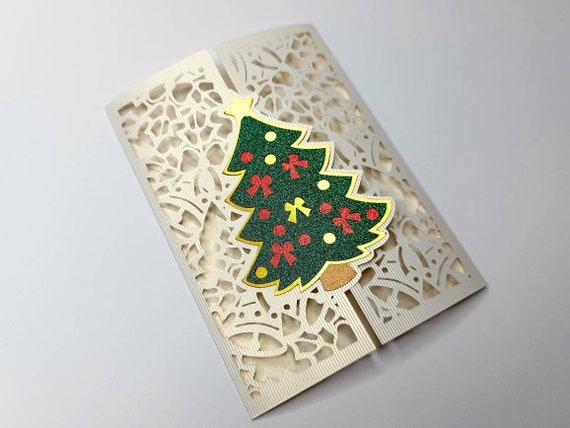In the photograph, a sophisticated Christmas card lies diagonally against a light medium gray background, with its bottom to the lower right of the frame and its top extending to the upper left. The card, primarily tan or white, features intricate cutout designs resembling bells, bows, and possibly other shapes. Its unique French door-style opening is indicated by a slit down the middle, suggesting it opens from the center. In the middle of the card, a beautifully adorned Christmas tree takes center stage. The green tree, with a textured surface, is outlined in gold or yellow and topped with a yellow star. It is decorated with red ribbons, along with gold and red baubles, and reveals a brown trunk. Inside, a smoother gold surface can be seen through the cutouts, adding to the card's elegant design.